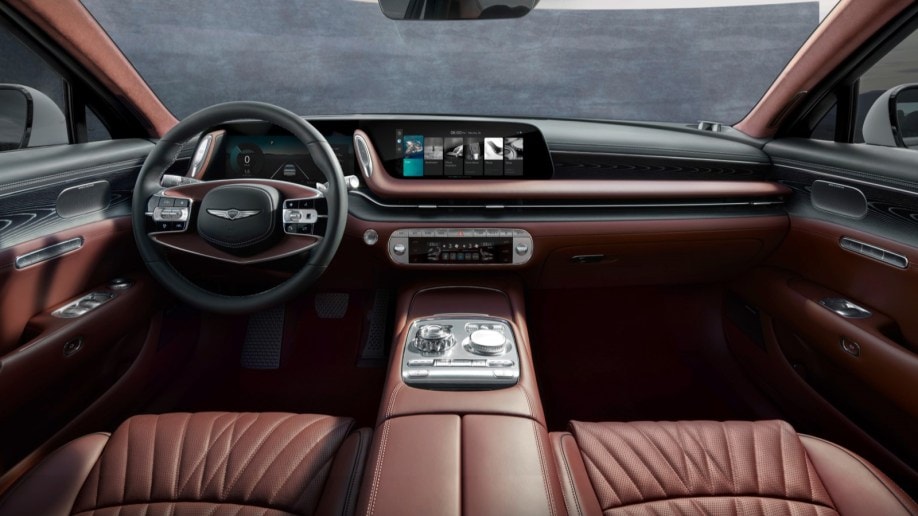The image captures the interior of a luxurious vehicle from a centered, forward-facing perspective. The interior exudes elegance, dominated by rich brown leather that adorns the seats, central console, and much of the side paneling and dashboard. The dashboard is primarily black, but features distinctive reddish-brown trims in the middle and at the very bottom. The console is also brown, with the exception of a silver section near the front, adjacent to the touchscreen and radio panel. The steering wheel is a striking black with a brown design in the center, embellished with several controls and a chrome winged brand symbol. The doors, fully in sync with the interior palette, are similarly trimmed in the same reddish-brown color. Through the windshield, a gray wall is visible, and the only hint of the car's exterior – the side mirrors – suggests a white exterior finish.